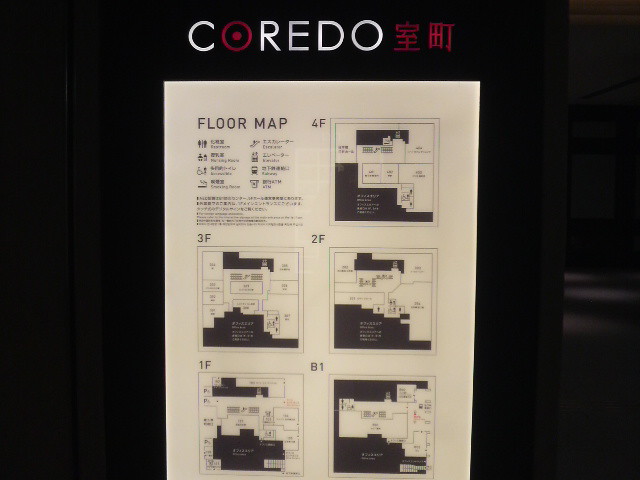This photograph displays a detailed floor map intended for navigating a mall, labeled prominently with "COREEDO" at the top, accompanied by Japanese characters. The map is printed on a white background and features a combination of English and Japanese text. It enumerates various floors of the mall, labeled as 4F, 3F, 2F, 1F, and B1, with each floor plan delineated in black and white. The plans include symbols indicating amenities such as bathrooms, handicap access, elevators, escalators, and even trains. Each floor’s layout is shown with small boxes representing different businesses, although the business names are slightly out of focus. Surrounding the map is a black backdrop, creating a visual contrast that emphasizes the white of the map. The text "COREEDO" also includes a distinctive red circle within the first "O" and is highlighted with additional red Japanese symbols to the right, giving the map a stylish and culturally specific design.